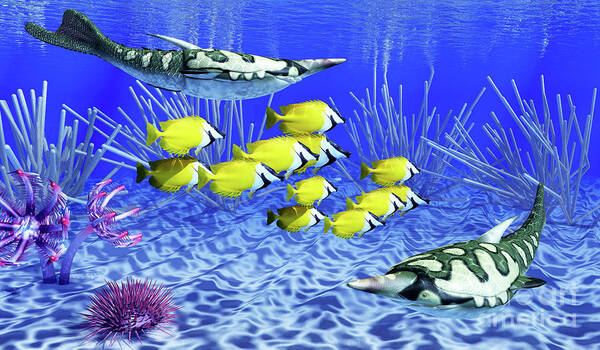This is an underwater photograph or possibly an aquarium scene depicting a vibrant ocean floor. The background is a vivid royal blue, accentuated by streaming sunlight and slight ripples on the water’s surface. Distinct coral structures dot the seafloor, including clear green, blue, and purple corals, as well as magenta aquatic plants. A purple sea urchin is nestled among the corals.

Central to the image is a school of small, yellow fish with black and white highlights around their heads, swimming toward the right. Above them, a prominent fish with a long, pointed nose, likely a swordfish, swims in the opposite direction. This fish has a white underbelly, a gray upper body with a textured pattern, and a dark gray tail. At the bottom right, another similar fish swims leftward, mirroring the first.

Amidst this aquatic tableau is a solitary angelfish with distinctive white stripes across its mouth and fins. The overall effect of the scene is reminiscent of a vibrant painting or computer-generated imagery, showcasing the vivid colors and dynamic movement typical of a lively underwater ecosystem.